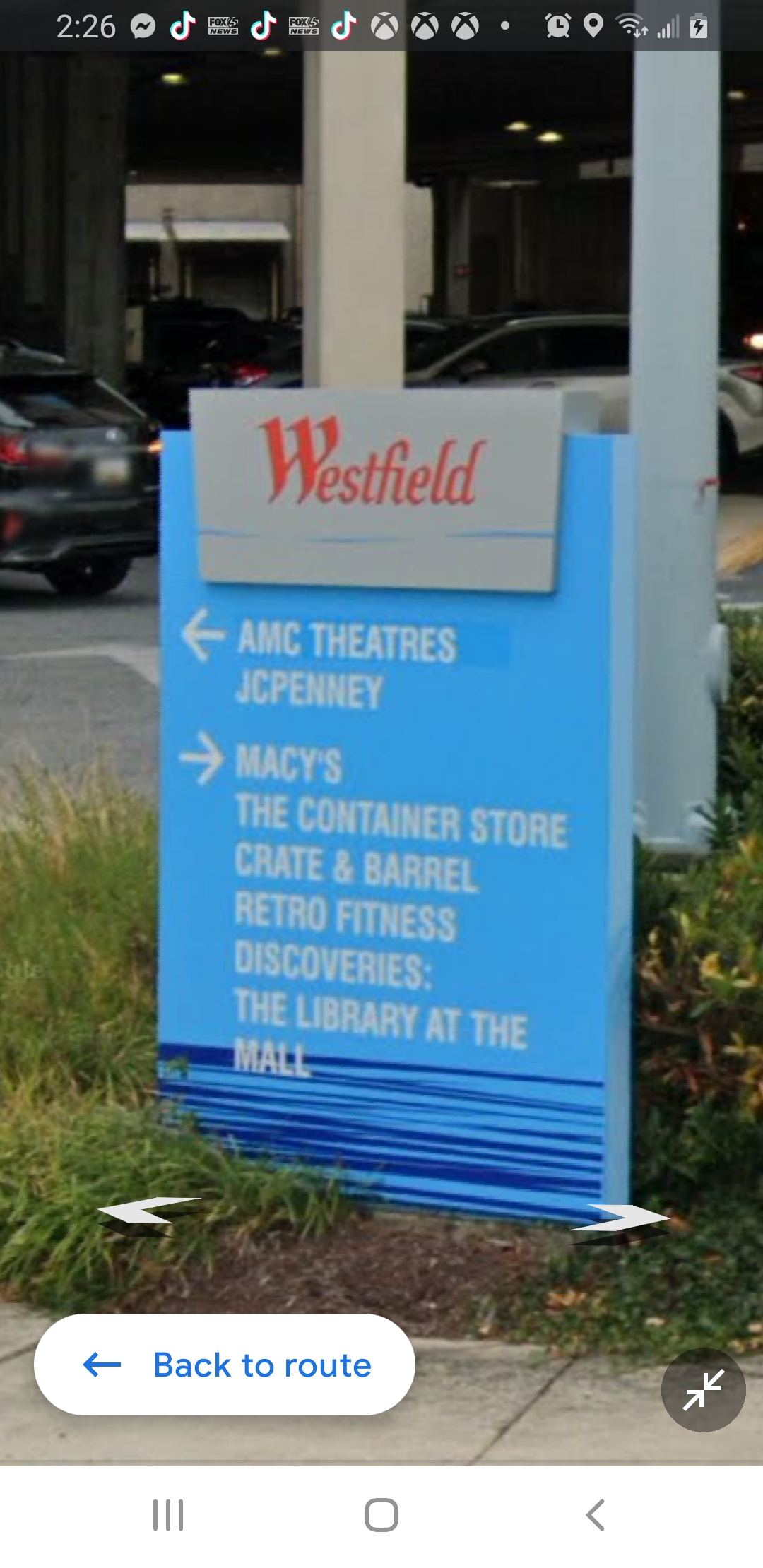The image captures a digital menu board at Westfield Mall, serving as an interactive directory similar to Google Maps Street View. The menu board is situated in front of a parking garage and is framed by tall grass. It features a light blue background with white, all-caps text.

Positioned at the top of the screen are various icons: the time (2:26), Facebook Messenger, TikTok, Fox News, Xbox (tentative identification), an alarm clock, a location symbol, a Wi-Fi icon with up and down arrows, signal carrier bars with three filled, and a battery icon indicating around 80% charge.

The top of the menu reads "WESTFIELD" in grey. Below, directional instructions are clearly displayed: a left arrow pointing to AMC Theaters and JCPenney; a right arrow guiding towards Macy's, the Container Store, Crate and Barrel, Retro Fitness, and Discoveries: The Library at the Mall.

In front and slightly beneath the menu board are interactive arrows typically found in street view interfaces, allowing users to change their view. At the bottom right corner, there is a circle with two white arrows in a point-to-point configuration and an oval labeled "Back to Route" in green with a left-facing arrow.

This detailed depiction showcases the mall’s technological engagement and user-friendly navigation aids.